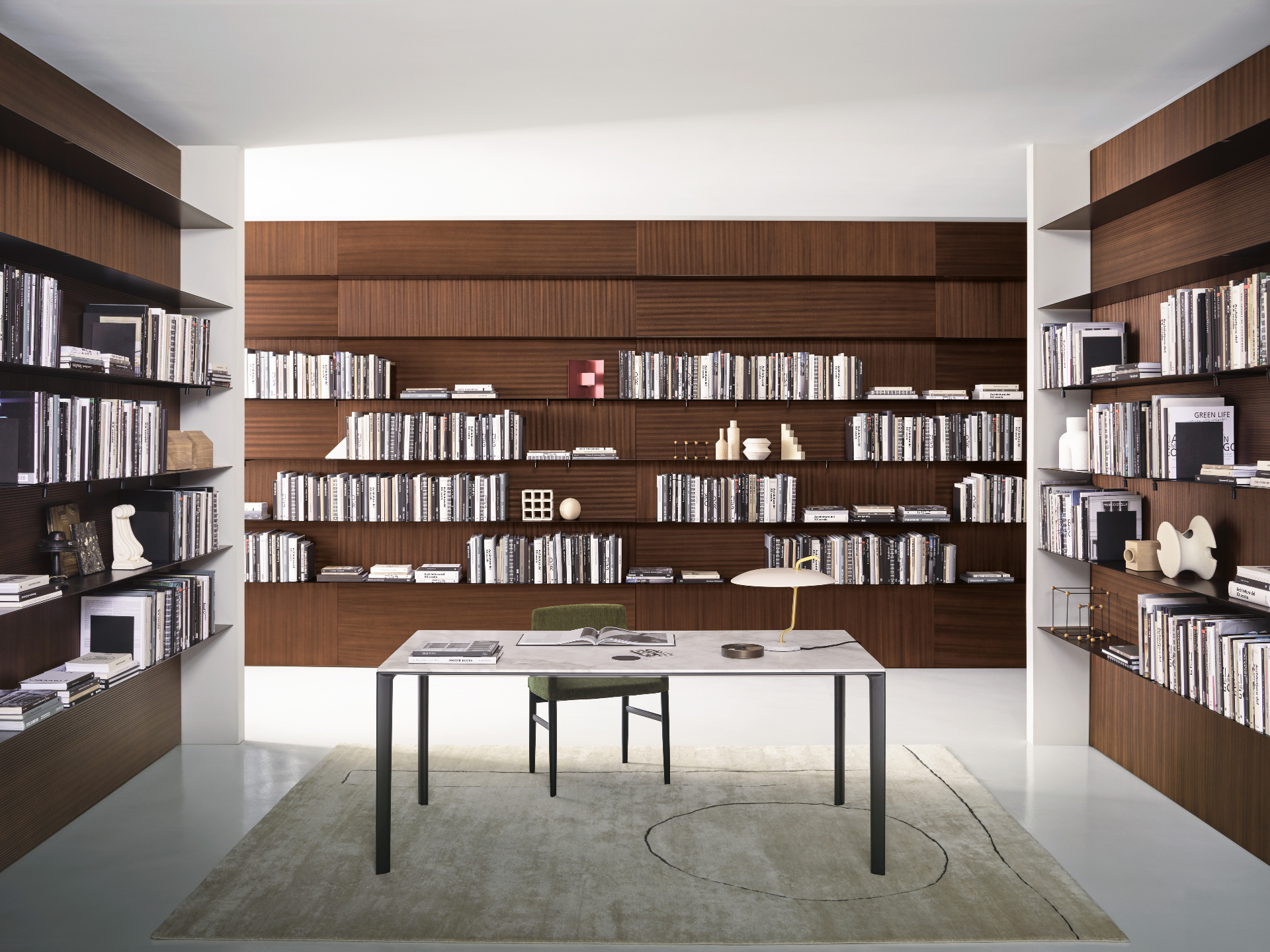This photograph depicts a modern, minimalist library or office space featuring a central table on a tan, geometric-patterned rug set against a white, tiled or linoleum floor. The table is white with black legs and is accompanied by an olive-green chair. Atop the table, there are several books, including an open one, assorted papers, and a striking white desk lamp with a brass base and support. The lamp emphasizes the room's sleek, modern aesthetic.

The room is surrounded by bookshelves crafted from a mahogany wood color, lining the walls on the left, right, and rear. These shelves are meticulously organized, holding an array of books both horizontally and vertically arranged, some with protective paper covers. The shelves also host various knick-knacks and ornaments, such as bookends, a set of miniature stairs, and a small decorative ball, adding a touch of personality to the space.

The ceiling is white, contributing to the room's bright and airy ambiance. The photograph, slightly longer than it is tall, captures the entire scene, highlighting the interplay between the minimalist furniture and the abundant, yet neatly arranged books and items on the wooden shelves.